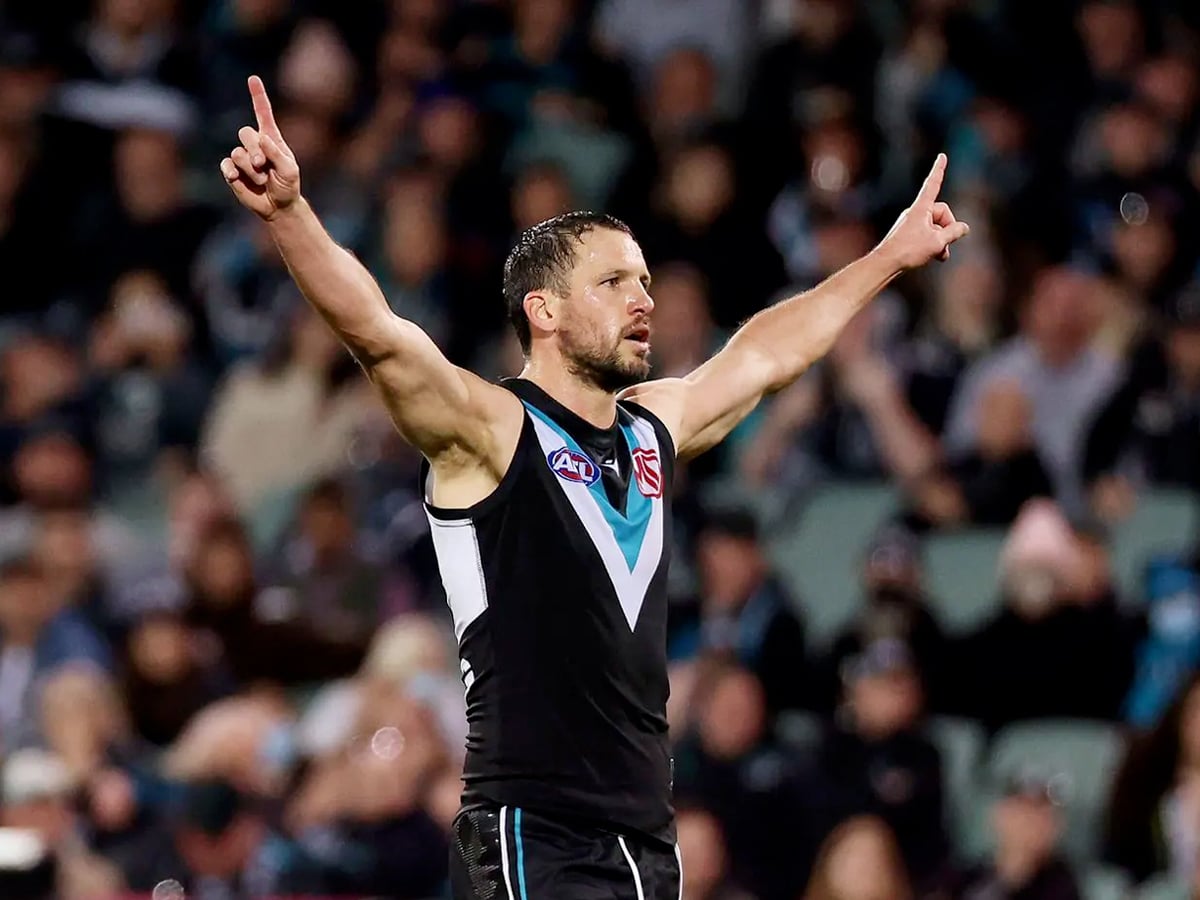The image showcases a close-up, high-resolution photograph of a Caucasian man, who appears to be a professional athlete, at the center of the frame. He stands with his arms outstretched straight up, his pointer fingers extended towards the sky. The man is dressed in a sleeveless black tank top featuring white and blue 'V' designs, and black shorts adorned with blue and white stripes. He has short, slicked dark brown hair, a dark mustache, and a beard. His expression conveys a look of surprise, and he appears sweaty, suggesting involvement in a physically demanding activity. The background is blurred, revealing a crowded audience seated in stands, enhancing the impression that this is a sporting event. The overall composition, combined with the man's athletic attire and demeanor, leads to a strong suggestion that the scene is from a high-stakes competition, possibly even an Olympic event.